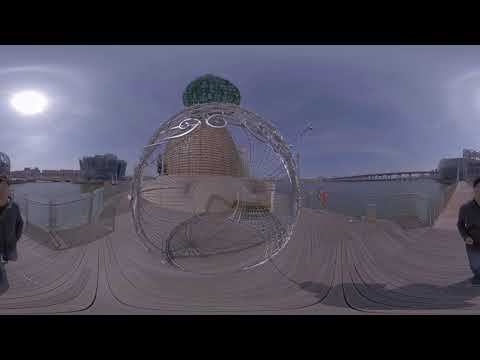The image captures a distorted panoramic waterfront scene under a purplish-blue sky. In the background, the sun appears pale and situated in the upper-left corner above a lagoon, which is bordered by a fence. The central focus is a large, cylindrical ornament that resembles a ring, seemingly out of place. Swirling, gray, wet sand dominates the foreground, contrasting with the grayer water nearby. On the right side, a pier extends into the water, with another pier visible further off in the distance. The sky, not very bright, lends a somber tone to the scene. Two instances of the same person, depicted due to the panoramic effect, are visible on both the right and left sides of the image, wearing a black long-sleeved top and blue jeans. Vertical lines resembling tire tracks are seen on the cement or asphalt surface. A bridge can be seen extending across the water in the far distance to the right, while tall, strange buildings loom on the left. The entire scene is overlaid with black bars at the top and bottom, suggesting it might be extracted from a video, resulting in an overall highly distorted, almost surreal representation of a waterfront area.